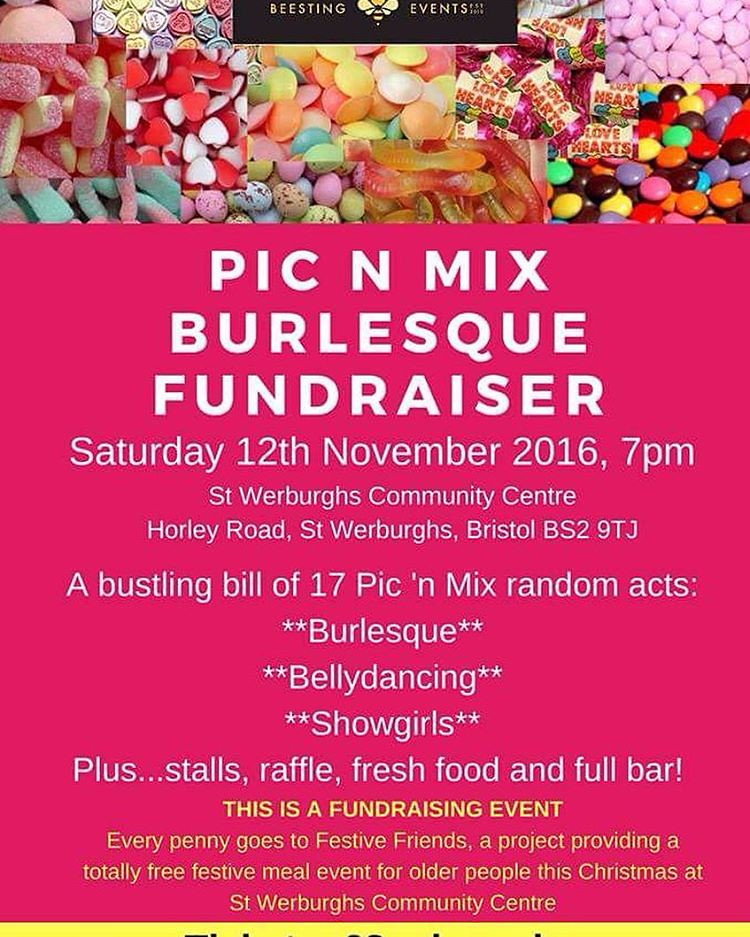**Advertisement Poster: Pick and Mix Burlesque Fundraiser**

At the top of this vibrant advertisement poster, a composite set of colorful candy images including love hearts, gummies, M&Ms, valentines, little valentines, dinosaur eggs, and various colored dots, forms the banner. Below, the main body of the poster features a hot pink background with large text in light pink and yellow.

The main event details are prominently displayed, announcing the "Pick and Mix Burlesque Fundraiser" scheduled for Saturday, November 12th, 2016 at 7 p.m. The venue is St. Weber's Community Center, located on Hawley Road, St. Weber's, Bristol, BS29TJ.

The poster promises a bustling bill of 17 pick and mix random acts, featuring burlesque, belly dancing, and showgirls. Additionally, there will be various stalls, a raffle, fresh food, and a full bar.

Highlighted in yellow text, the poster emphasizes that this is a fundraising event with every penny going to Festive Friends, a project dedicated to providing a totally free festive meal event for older people this Christmas at St. Weber's Community Center.